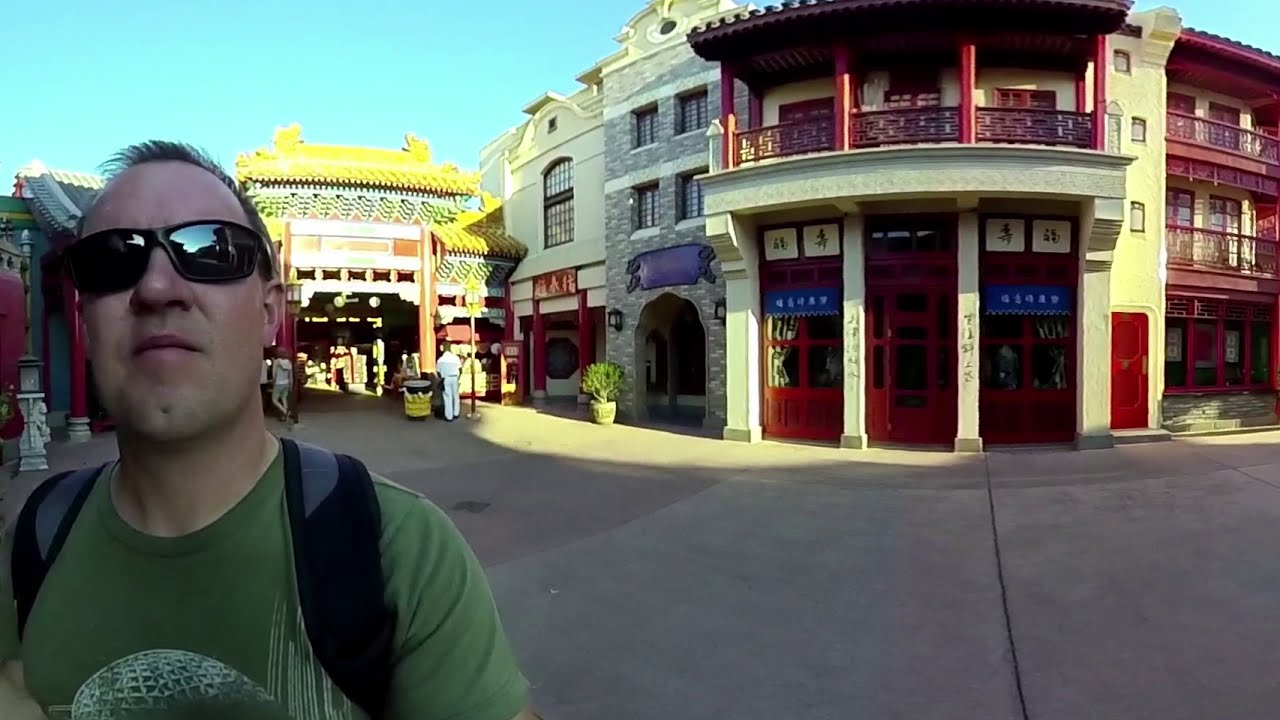This image captures a vibrant street scene in an Asian city, most likely China, during a sunny daytime with a clear, light blue sky. Dominating the background is a multi-story building featuring traditional Asian architecture, characterized by red doors and windows, topped with a gold gabled roof adorned with intricate carvings and possibly dragon motifs. The second floor of this building has a balcony supported by red pillars, with Chinese characters displayed on white signs mounted on the posts.

In the bottom left corner of the photograph stands a middle-aged man with short hair, wearing a kelly green graphic t-shirt depicting a globe-like emblem on the front. He has black and gray backpack straps over his shoulders, black rimmed sunglasses with reflective lenses, and a distinctive dimple on his chin. He appears to be looking upwards, away from the camera.

Surrounding this focal building are other structures, ranging from gray stone to white concrete, some sporting Asian characters in red and blue. Below the buildings, the pavement is dotted with pedestrians, one notably moving buckets, and there's also a black garbage can with yellow markings. Despite the urban bustle, the man in the foreground appears shaded, adding a contrast to the sunlit background.